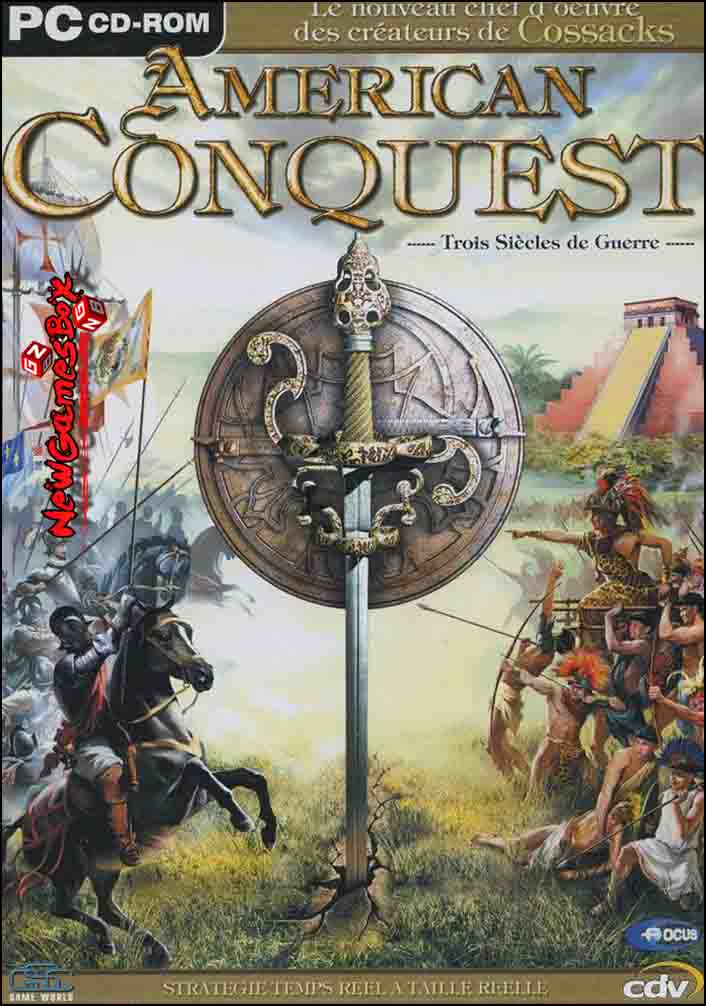The image is a vertical, rectangular computer game cover for "American Conquest" with a clear "PC CD-ROM" label at the top left corner. Dominating the center is a visually striking dark golden-brown metal shield with intricate carvings, positioned behind a massive, elaborately designed sword. The sword, featuring a skull at the handle's top and a gold snake winding around its grip, pierces the ground, causing it to crack dramatically. Flanking the central weaponry, the left side depicts armored soldiers on horseback, emerging from ships with white sails marked by crosses. Meanwhile, the right side presents indigenous warriors equipped with bows and arrows, set against the backdrop of a stepped pyramid with a golden ramp. At the cover's bottom, titles and logos such as "strategic temps réel atelier," "CDV," and "Same Game World" are visibly placed, adding to the historical and epic theme of the game.